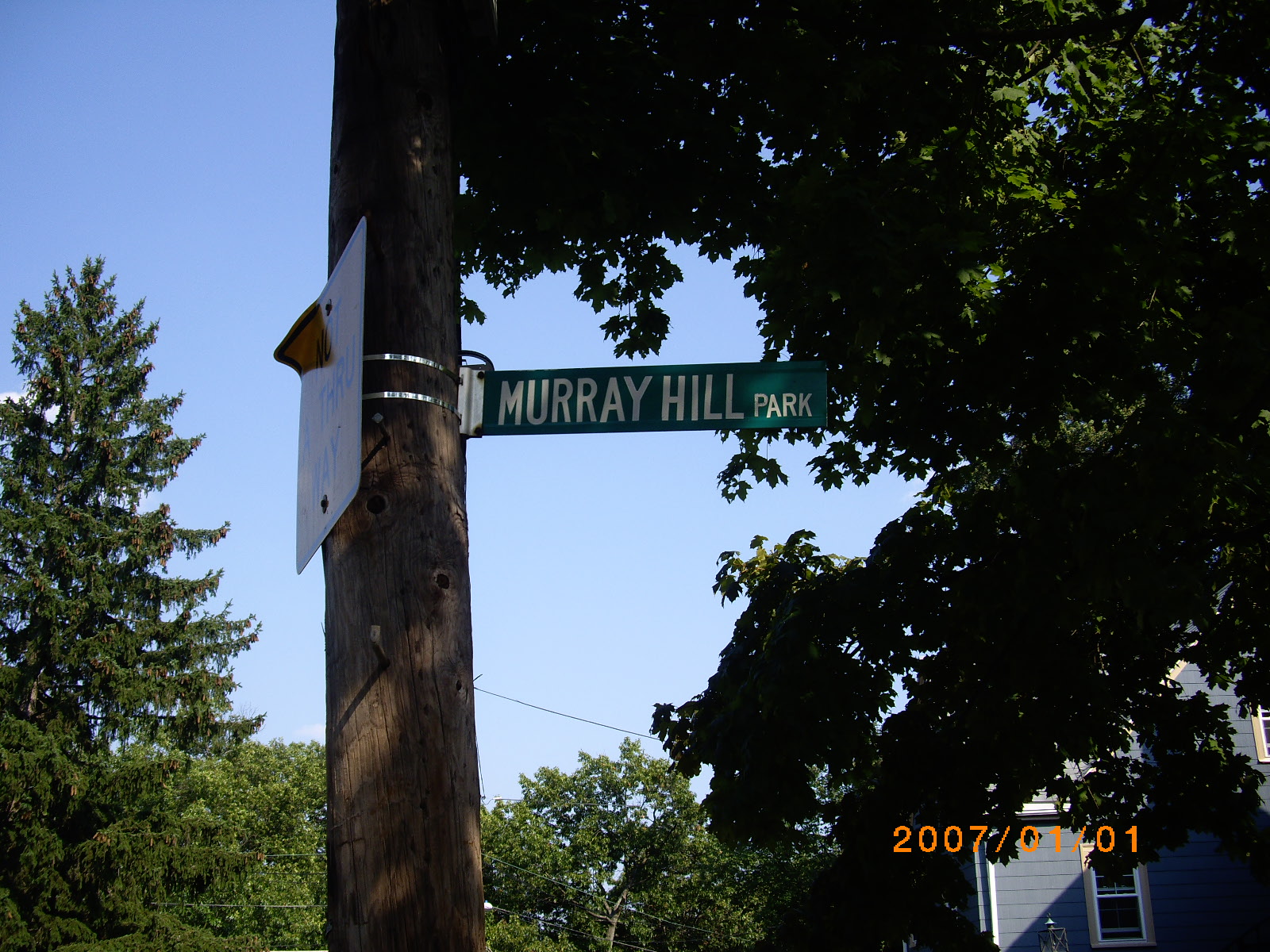The photograph captures a dark brown pole, which could be a telephone or electric line pole, prominently featuring a green street sign that reads "Murray Hill Park" in white letters. An additional sign is mounted on the backside of the pole but is not visible. At the bottom right corner of the image, the date "2007-01-01" is clearly displayed. In the background, to the right of the pole, a large, tall tree with green foliage stands out against a bright, medium blue sky devoid of clouds. Below the tree, a small blue house with white trim is partially shaded by the surrounding greenery. The scene is set on a sunny day, with sunlight casting on the house and trees, enhancing the natural colors. The greenery from various trees and a bush extends across the bottom and sides of the photo, stitching together a vibrant, outdoor setting.